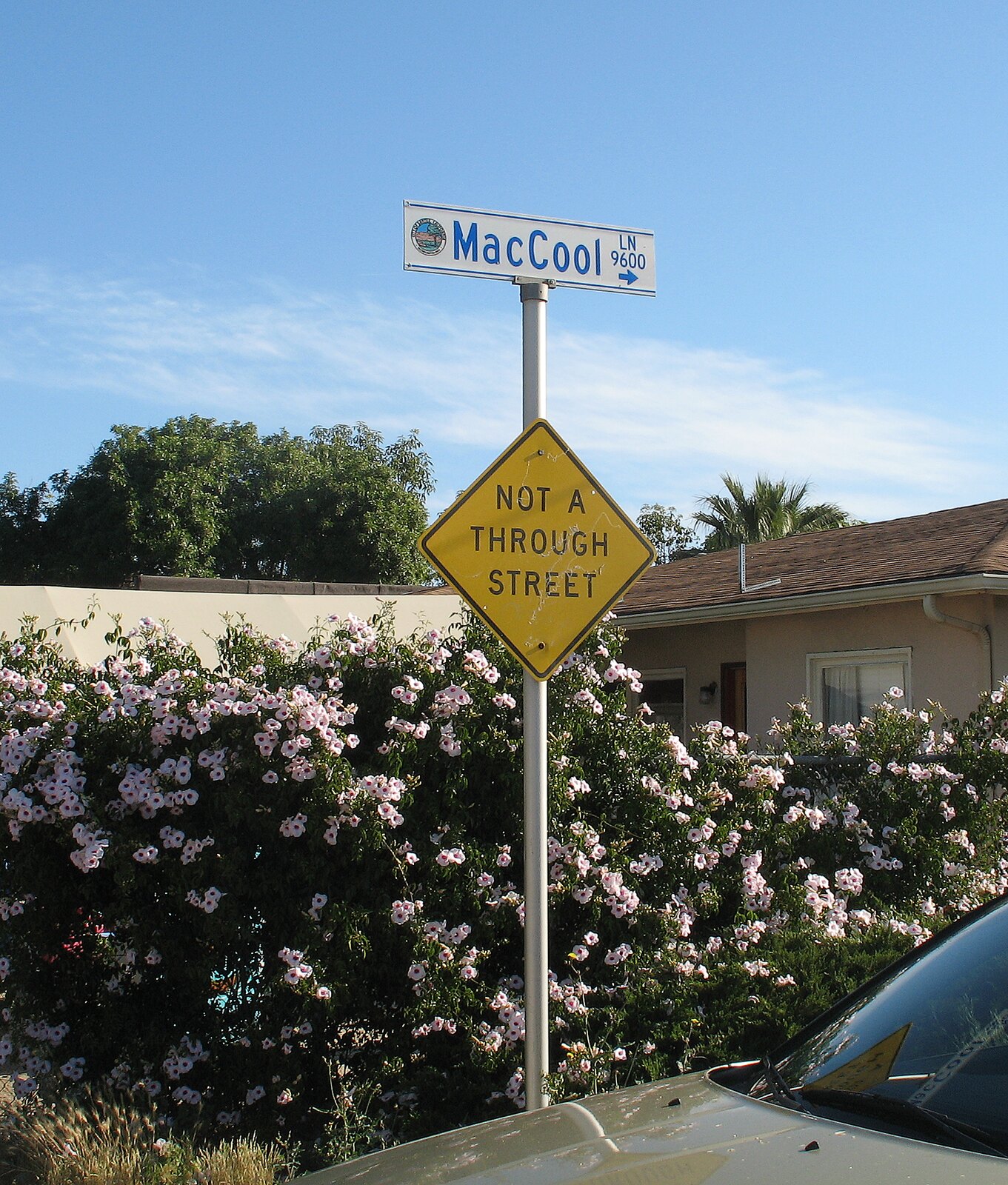In this vibrant daytime photograph, the foreground features a gold-colored vehicle prominently displayed. Standing behind the car is a metal pole bearing two signs; the lower sign has a striking yellow and black combination with the words "Not a Through Street" inscribed in bold black font. Above it, a blue and white sign reads "Mac Cool" along with letters, numbers, and an arrow directing towards a specific location. Directly behind the pole, a lush green bush adorned with delicate, pale pink flowers adds a splash of natural beauty to the scene. Further back, a tan-colored house capped with a brown roof is partially visible, surrounded by verdant trees. The backdrop is completed by a clear blue sky accentuated with wispy clouds, contributing to the overall serene atmosphere.